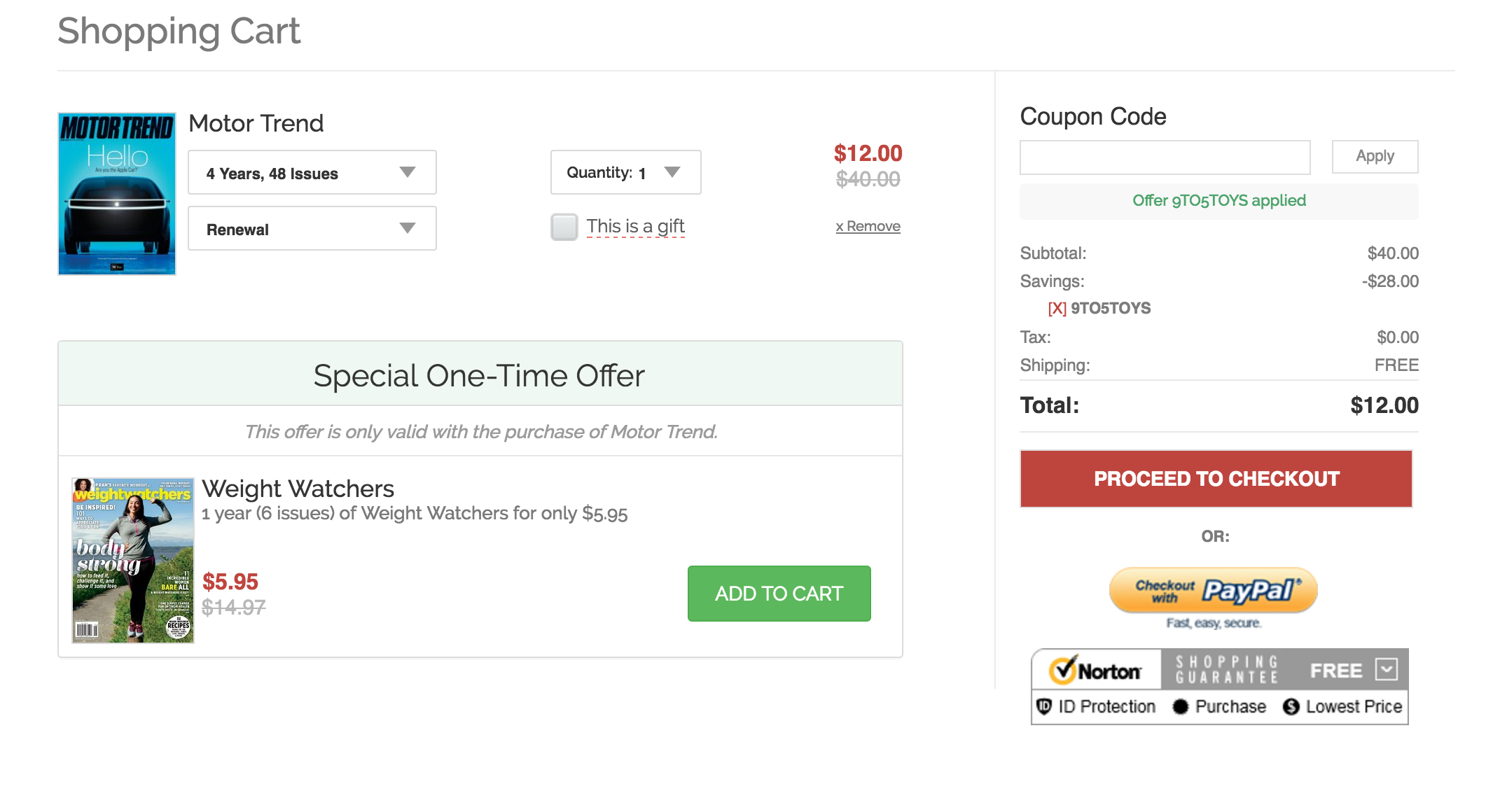Detailed Caption:

This image captures a detailed view of an online shopping cart interface. In the top left corner, gray text prominently designates "Shopping Cart." Below, a featured image shows a car with the title "Motor Trend" displayed above it in large text. Underneath the image, in white text, it says "Hello," and in smaller black text, it repeats "Motor Trend." Adjacent to this is a dropdown menu offering subscription options; the default selection shows "Four Years, 48 Issues, Renewal," suggesting that Motor Trend is a magazine subscription.

To the right of this option, the quantity is listed as "1," with an adjacent checkbox allowing users to mark it as a gift. The item is priced at $12, down from $40, with an option to remove it from the cart.

Below, there is a promotional offer featuring the "Weight Watchers" magazine. A small cover image of the magazine is displayed, with text indicating a special offer—one year (six issues) for $5.95, discounted from $14.97, alongside an "Add to Cart" button for this offer.

Further down the page, the cart summary is provided. Users can enter and apply a coupon code in the designated field. The breakdown includes a subtotal of $40, savings of $28, zero tax, and free shipping, culminating in a total of $12. Below the total, two buttons offer checkout options: a red button with white text labeled "Proceed to Checkout" and a yellow button with the PayPal logo for a PayPal checkout option. Lastly, an icon at the bottom signifies that the transaction is protected by Norton Security.